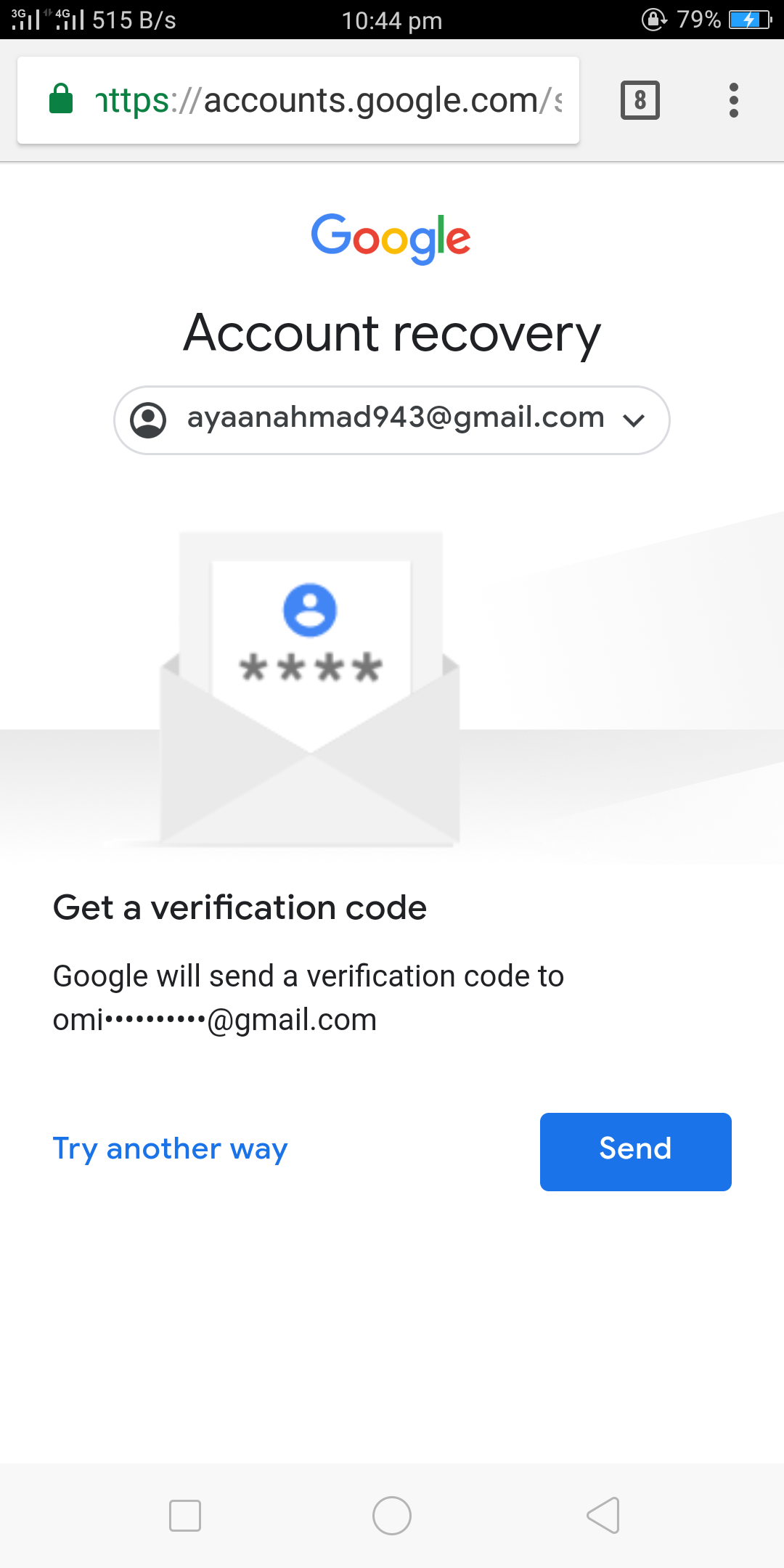Screenshot Description: 

The image is a screenshot taken from a mobile device showing a webpage. At the very top of the screen, there is a black notification bar. On the left side of this notification bar, there are two icons indicating data signals, with the first one unclear, and the second one displaying "4G" with a data rate of "515B/s" next to it. The current time is shown in the middle as "10:44 PM", and on the right side, the battery level is indicated to be at "79%".

Below the notification bar, an address bar is visible, showing the URL "accounts.google.com". Next to the URL, on the right side, there is a square icon with the number "8" inside it, indicating that eight pages are open.

The content of the webpage centers around Google Account Recovery. The word "Google" is prominently featured at the top center of the page. Beneath this, the phrase "Account recovery" is displayed. A text input field follows, where a username has been entered.

Below the input field, there is an icon of an open envelope with a piece of paper protruding from the top. The paper has a blue circle with four blue stars underneath it. The text below this icon reads, "Get a verification code. Google will send a verification code to OMI****@gmail.com."

At the bottom of the screen, on the left side, there is a clickable option that says "Try another way". On the right side, a blue "Send" button is prominently displayed.